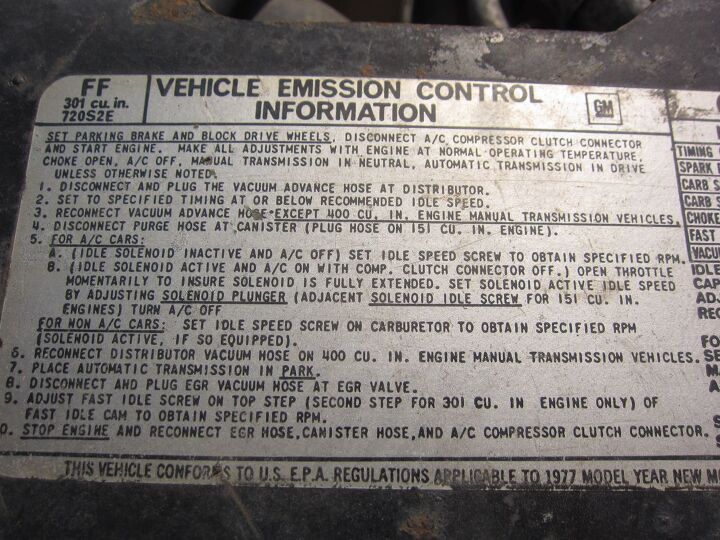The image features a close-up of a worn and dirty vehicle emission control information sticker, likely affixed to a rusted component of an old motor vehicle. The background of the sticker is white or silvery gray, with extensive text printed in black. Dominating the top right corner is a small, square "GM" logo representing General Motors. The largest text on the sticker reads "Vehicle Emission Control Information." To the left of this title, it lists "FF 301 cubic inches 720 S2E," possibly referencing engine specifications or serial numbers. The sticker is crowded with detailed instructions, including a numbered list from 1 to 10 with steps for setting the parking brake, blocking drive wheels, and various adjustments for different vehicle configurations. Key phrases are underlined, providing specific instructions such as "set parking, brake and block, drive wheels," and other mechanical adjustments. At the very bottom, the sticker confirms that the vehicle complies with U.S. EPA regulations for the 1977 model year. The focus of the image is solely on the sticker, with no other elements captured in the frame.